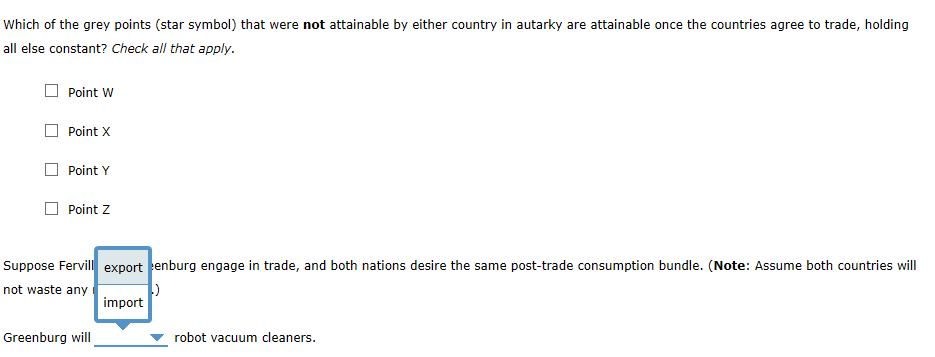The image is a screenshot displaying a white background, with no visible details indicating the source website. At the top of the screenshot, there is a question written in a medium gray font. The question reads: "Which of the gray points (*) that were not attainable by either country in autarky are attainable once the countries are able to trade, holding all else constant? (Check all that apply.)"

Below the question are four possible answers:
- Point W, with a gray checkbox to its left
- Point X, with a gray checkbox to its left
- Point Y, with a gray checkbox to its left
- Point Z, with a gray checkbox to its left

Beneath these options is the beginning of another sentence that starts with "Suppose," but the rest of the sentence is obscured by a pop-up menu. The partially visible text states: "Suppose [country name] engage in trade and both nations desire the same post-trade consumption bundle. (Assume both countries will not waste any...)"

The pop-up menu partially obscuring the text is a small rectangle. The top half of the rectangle has a light blue background and the word "export" in black, while the bottom half has a white background with the word "import."

The sentence partially obscured by this pop-up menu begins with "Greenberg will," followed by a dropdown menu symbol (a small inverted triangle) next to "robot vacuum cleaners." This implies a choice for the user to select whether "Greenberg will import robot vacuum cleaners" or "Greenberg will export robot vacuum cleaners," and the user is required to make the correct selection.